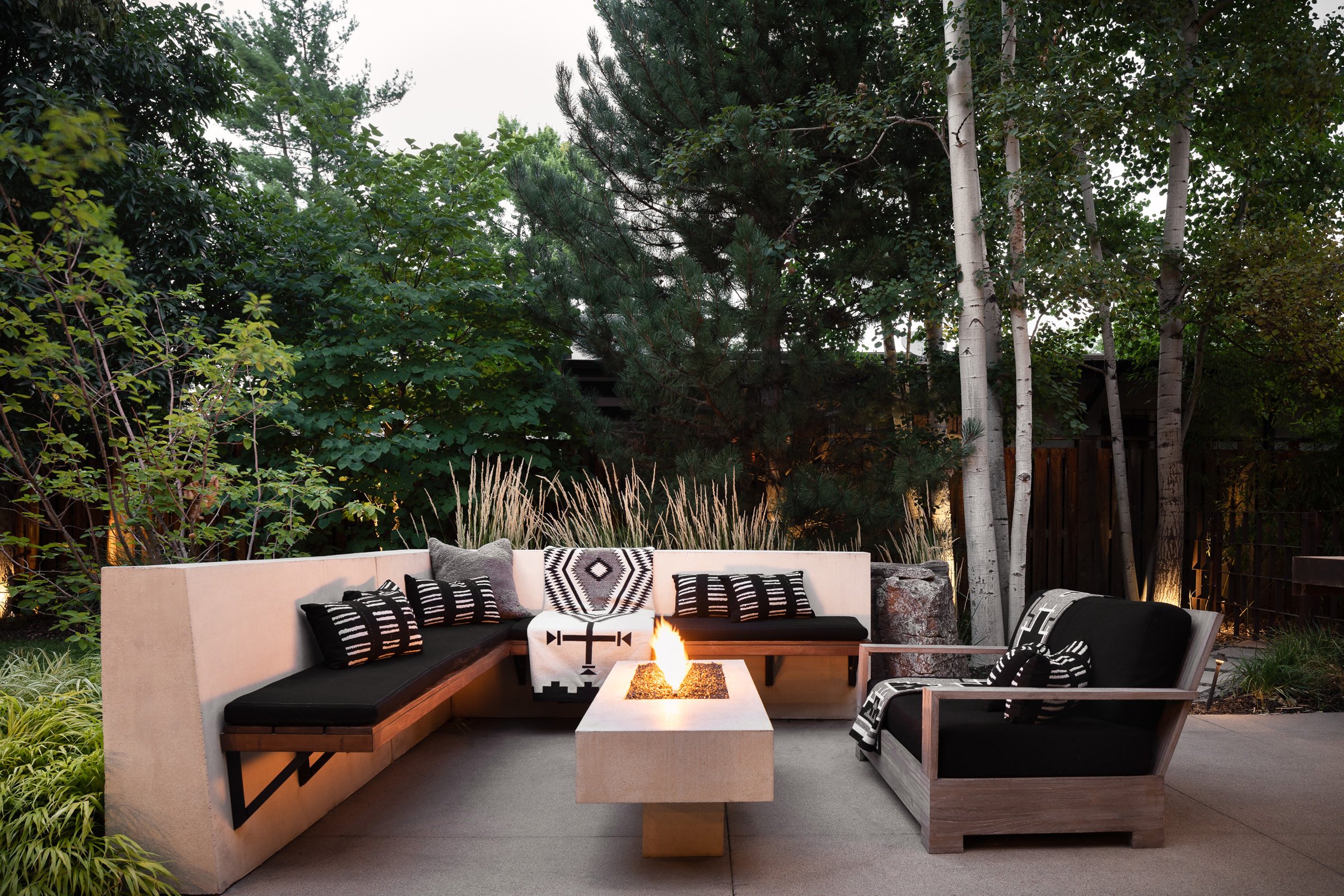The photo is of a beautifully decorated outdoor patio surrounded by lush trees, green foliage, and white birch trees. The patio floor is made up of light gray concrete slabs. Against a beige concrete wall on the left, there is an L-shaped wooden bench with black cushions, adorned with black and white striped pillows, and a black and white blanket draped over one side. To the right, there's a wooden love seat with black cushions and a similar blanket. In the center of the patio, there's a rectangular fire pit with a concrete body and a wooden base, emitting a leaping flame. Beyond the patio, there's a tall privacy fence and a pathway, with another house visible in the background under an overcast sky. The whole setting combines comfort and style, creating a cozy and inviting outdoor space.